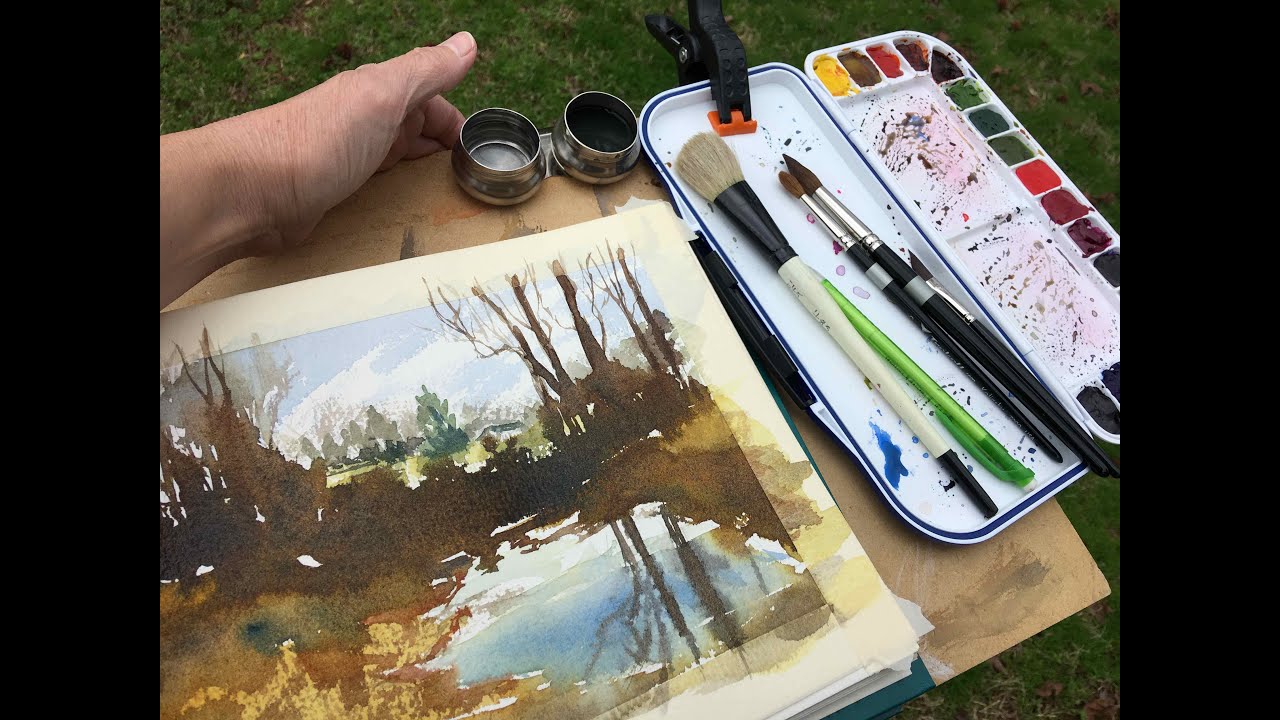In the foreground of this detailed image, a human hand emerges from the perspective of the camera, firmly gripping a wooden plank upon which a scene lies meticulously arranged. Front and center on the plank is a watercolor painting rendered on cream-colored paper, capturing a serene forest scene surrounding a placid, reflective lake. The forest is characterized by dark brown trees and light brown grasses, while the pond boasts a brilliant blue, mirroring the woodland around it.

To the right of the painting rest two small plastic containers. One is a compact clamshell case dedicated to the artist's paintbrushes and paints. The open clamshell reveals four paintbrushes: two with black handles and fine tips, one with a green handle and an extremely fine tip, and one with a white handle and a broad tip. The other side of the clamshell features several trays each holding a different watercolor paint. 

Also on the wooden plank, aligning with the top, are two small tins which likely serve as water cups or additional storage for essential painting supplies.

The entire composition, set against a background of lush green grass, epitomizes an artist's workspace.